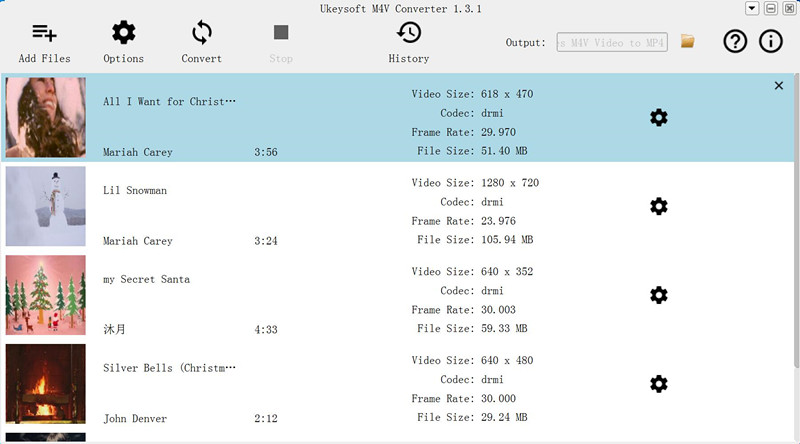In the image, a software interface with a gray background is presented. At the top of the interface, a series of black icons are displayed, each representing different functions: Add Files, Options, Convert, Stop, History, and Output. Centrally placed at the very top in the same gray background is the title "UKeysoft M4V Converter 1.3.1."

Below this header, there is a white background area. On the left side of this section, there are colorful thumbnails representing different videos. Next to each thumbnail is the video's title, duration, and file size. Further to the right, each entry has a gear icon, indicating settings options for individual videos.

The videos listed include:
1. **"All I Want for Christ" by Mariah Carey** - Thumbnail shows an image of Mariah Carey. The time is 256 seconds.
2. **"Lil' Snowman" by Mariah Carey** - Thumbnail features an image of a snowman. The time is 324 seconds.
3. **"My Secret Santa"** - Thumbnail depicts Christmas trees against a pink background. The time is 433 seconds.
4. **"Silver Bells, Christmas" by John Denver** - Thumbnail showcases a fire in a fireplace. The time is 212 seconds.